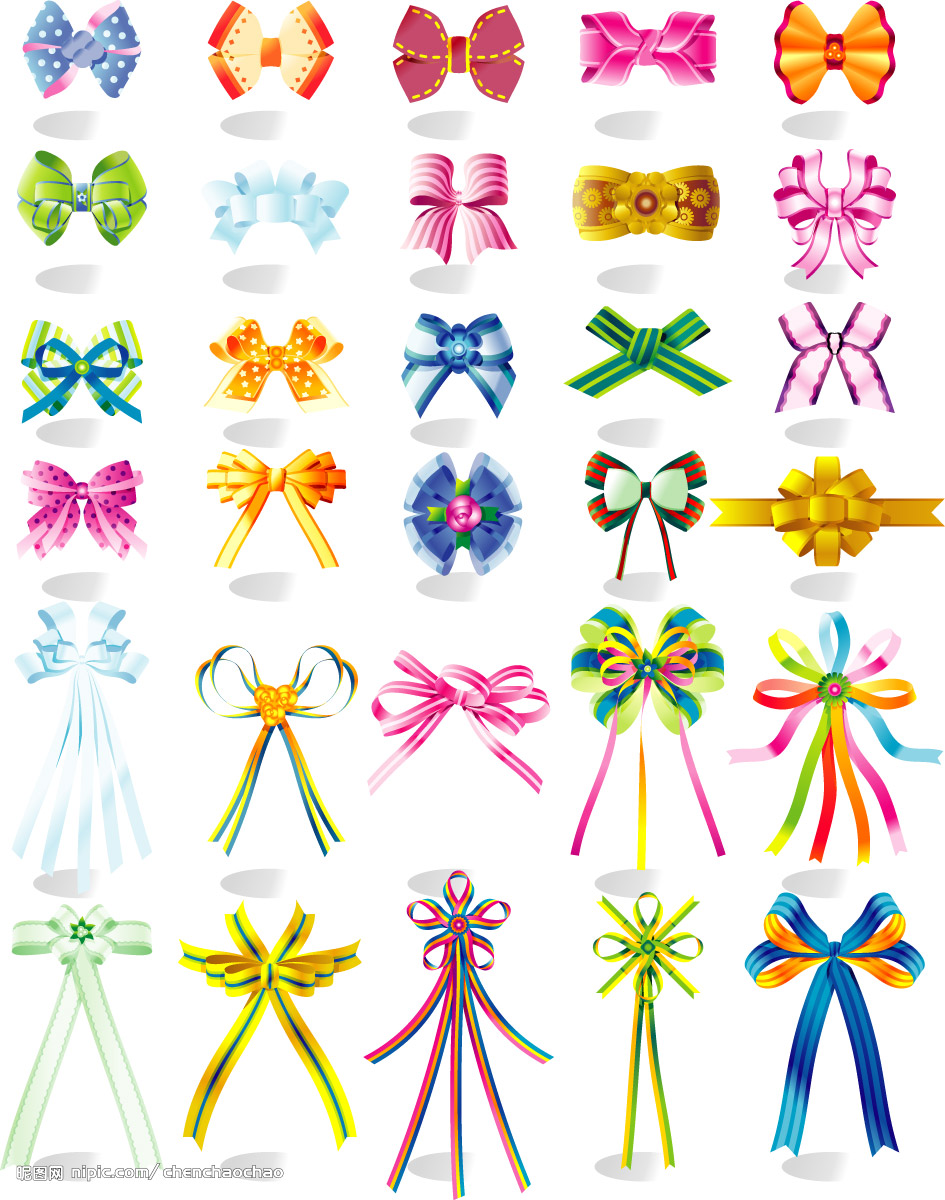This image is an educational poster showcasing a variety of 30 different bows and bow ties, arranged in a grid of five columns and six rows. Each bow is intricately illustrated to display the wide range of styles you can create, perfect for either wearing as a bow tie or using as decorative ribbons on packages. The bows vary in color, including vibrant greens, pinks, purples, blues, oranges, yellows, and multi-colored designs. Some bows feature patterns such as polka dots and look like ribbon candy in festive colors of green and red. Next to each bow is a small gray circular disc, possibly indicating the type of ribbon used. The poster also includes Asian text and a reference to the website nipic.com, under the username chenchaochao. This detailed and colorful guide makes it ideal for those in customer service packaging or anyone interested in crafting and learning different bow-tying techniques.